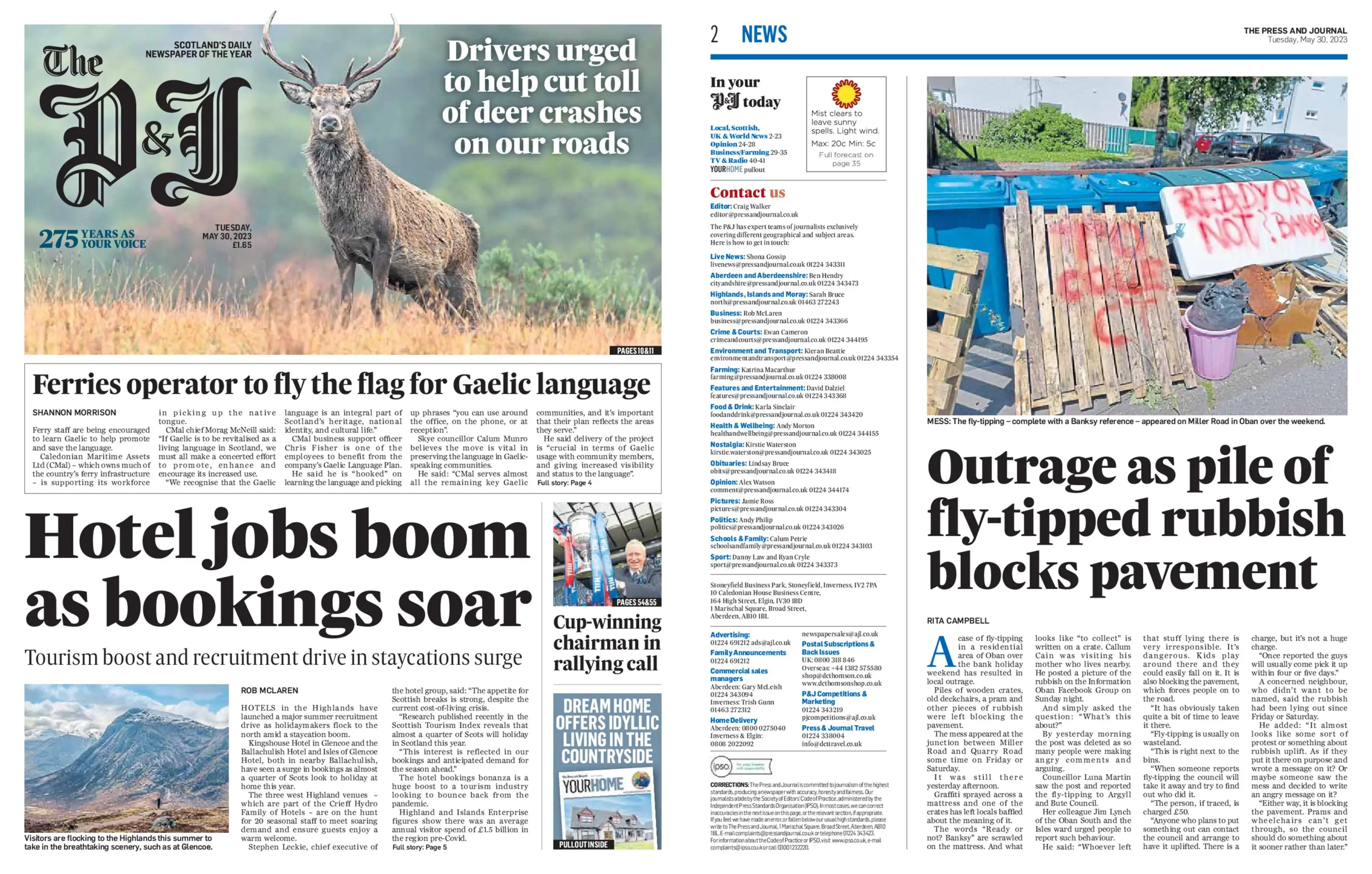Displayed on the screen are two pages from Scotland's renowned Daily Newspaper of the Year, The Press and Journal (PJ). The front page, dated Tuesday, May 30, 2023, features a striking photograph of a buck in a field alongside the headline, "Drivers Urge to Help Cut Toll of Deer Crashes on Our Roads," marking 275 years of the publication being "Your Voice." 

On the right side of the screen is page two, also from the same date, indicated by the numeral "2" and labeled "News." The prominent headline here reads, "Hotel Jobs Boom as Bookings Soar," reflecting the main story of increased employment opportunities in the hotel industry. Additionally, another significant story on this page captures public outrage with the headline, "Outrage as Pile of Fly-Tipped Rubbish Blocks Pavement," addressing the issue of illegal waste disposal obstructing pedestrian walkways.